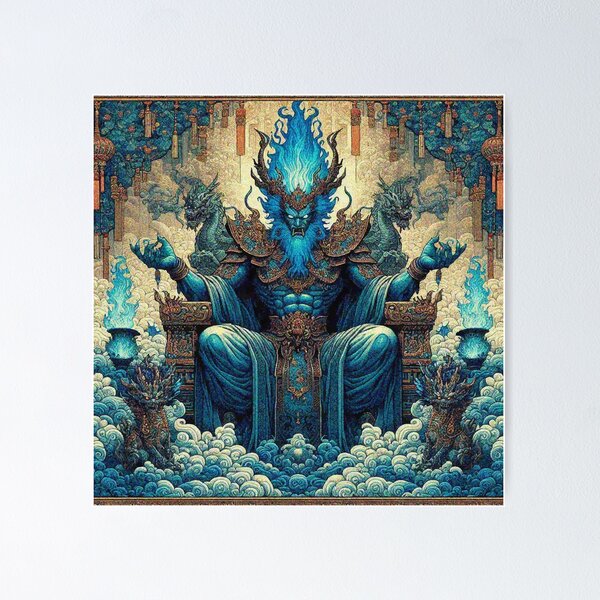This detailed drawing exhibits a Gothic, futuristic fantasy scene, akin to visuals from video games, potentially appealing to children. Centering the 4-inch square image with a light gray border and additional pinstripe and brown border accents, is a formidable and fierce character seated on a substantial, intricately carved stone throne. This imposing figure combines human and dragon characteristics, boasting a muscular, Schwarzenegger-esque build with blue-skinned arms and body. His dragon head features sharp fangs, white eyes, a blue beard, and blue flames emanating from his head, paired with horn-like projections forming a crown. Adorned in iron shoulder pads, from which green dragons protrude, and wearing a rusty armor belt and shoulder plates, his exposed torso and clawed hands resting on the armrests convey a sense of danger and malevolence.

Surrounding this central figure are oriental-style swirling clouds in hues of white, blue, and brown, adding to the fantastical ambiance. At the character's feet lie additional dragons, resembling dog-like creatures with dragon heads, while blue-flamed torches on either side contribute to the eerie atmosphere. The backdrop is illuminated by sunlight, enhancing the mystical environment, and decorated with hanging gold and orange bells. This image masterfully blends elements of gothic horror, fantasy, and oriental mystique, crafting a richly detailed and captivating visual narrative.